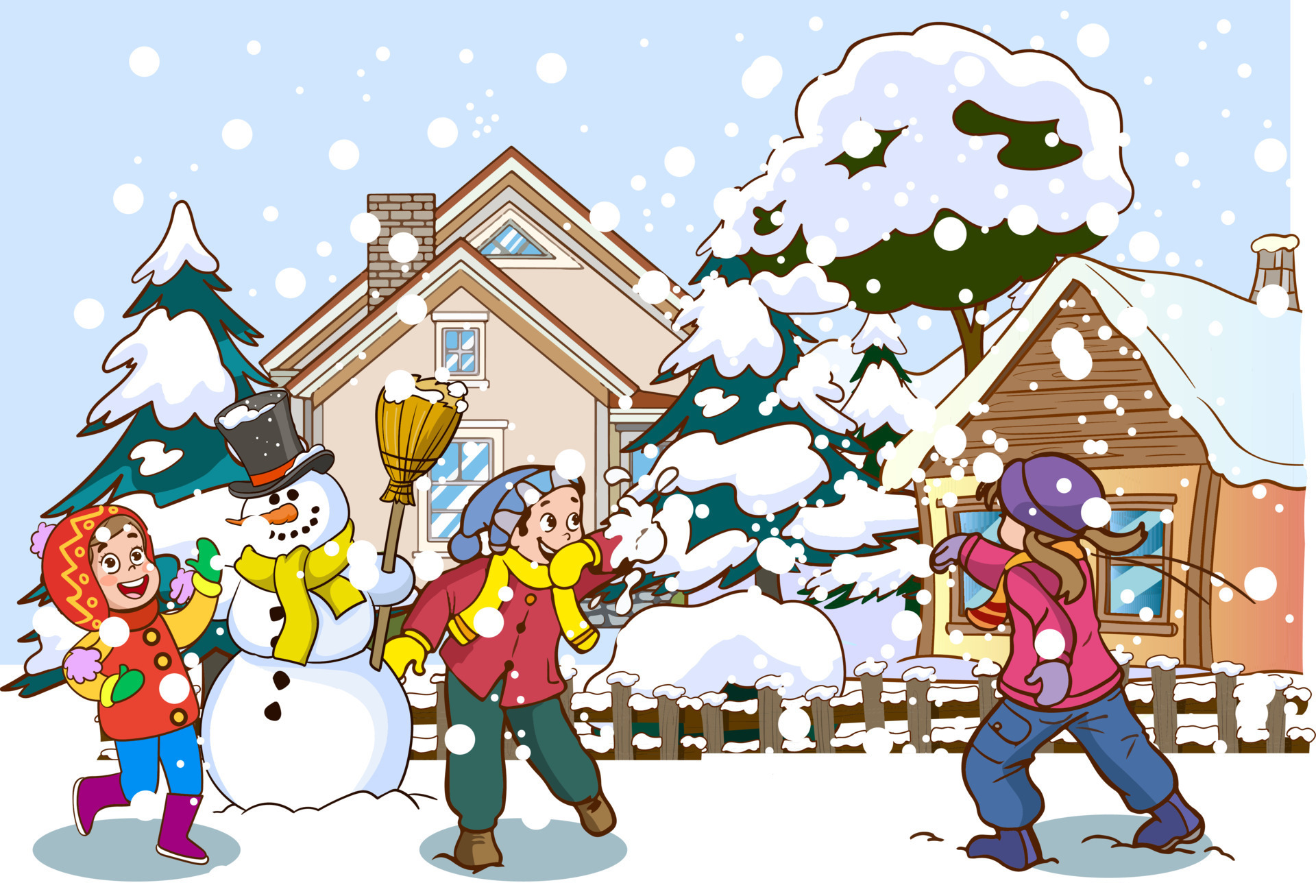This whimsical illustration, reminiscent of a classic Highlights seek-and-find picture, captures a delightful winter scene filled with youthful joy. In the foreground, three friends are exuberantly playing in the snow. To the right, a girl adorned in a red hat with yellow designs, a red shirt with yellow buttons and sleeves, green mittens, blue pants, and purple boots beams brightly as she enjoys the snowy day. Beside her stands a charming snowman, complete with a black hat sporting a red band, a yellow scarf, a carrot nose, two coal eyes, a wide smile formed by buttons, and four buttons down his front. His right arm, possibly wearing a glove, extends outward while his left arm holds a broomstick.

Adjacent to the snowman on the left, two children engage in a spirited snowball fight. The boy, donning a purple-blue hat, is captured mid-laughter as he blocks a snowball aimed at his face with his left arm. His cheerful attire includes a red jacket, yellow scarf, yellow mittens, green pants, and brown boots. Opposite him, a girl with a purple hat and brown pigtails is seen from behind as she prepares to throw a snowball. She wears a pink jacket, purple mittens, an orange and red scarf, blue pants, and blue boots.

In the background, two houses provide a cozy backdrop. The house on the right is tan with a red peaked roof, featuring an addition that juts out on the first floor. This house appears to have contrasting heights, possibly indicating a two-story section and a three-story section, complete with a prominent chimney. A snow-covered fir tree stands nearby, adding to the wintry atmosphere. To the left, another house with a snow-covered roof, wooden front framing, orange siding, and two front windows complements the scene. Snow-laden fir trees and delicate snowflakes falling from a clear blue sky complete this picturesque moment, making it feel like a charming illustration from a children’s magazine.